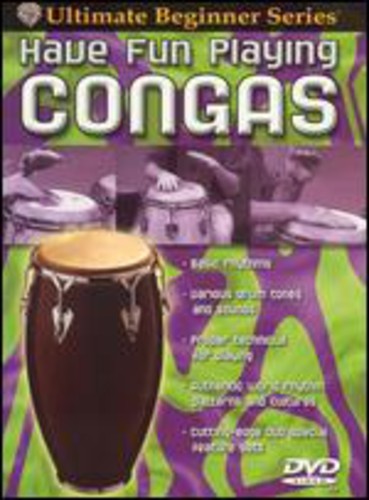The image above appears to be the cover of a DVD, characterized by a colorful and somewhat abstract design. Dominating the top of the cover is a black banner that reads "Ultimate Beginner Series" in yellow text. Directly below this, large white capital letters announce "Have Fun Playing Congas." The background behind this text features a vibrant swirl of green and purple hues, which continues towards the bottom of the cover, setting a lively tone. 

The bottom left of the DVD cover prominently shows a brown conga drum with a matching brown top, further emphasizing the musical theme. Beneath the main title, the cover is adorned with three images of people playing congas, all dressed in black shirts, with the middle figure possibly wearing white or blue pants. These images have a light purple background and appear to represent either three different individuals or multiple shots of the same person.

In the bottom right corner, the DVD logo is clearly displayed: a white oval with the letters "DVD" in bold white font inside it. Additionally, there is some blurry white text next to purple bullet points on the right side of the cover, though the text is unreadable. Despite the slight blurriness, the overall composition and vivid colors of the cover effectively communicate its instructional and engaging nature.